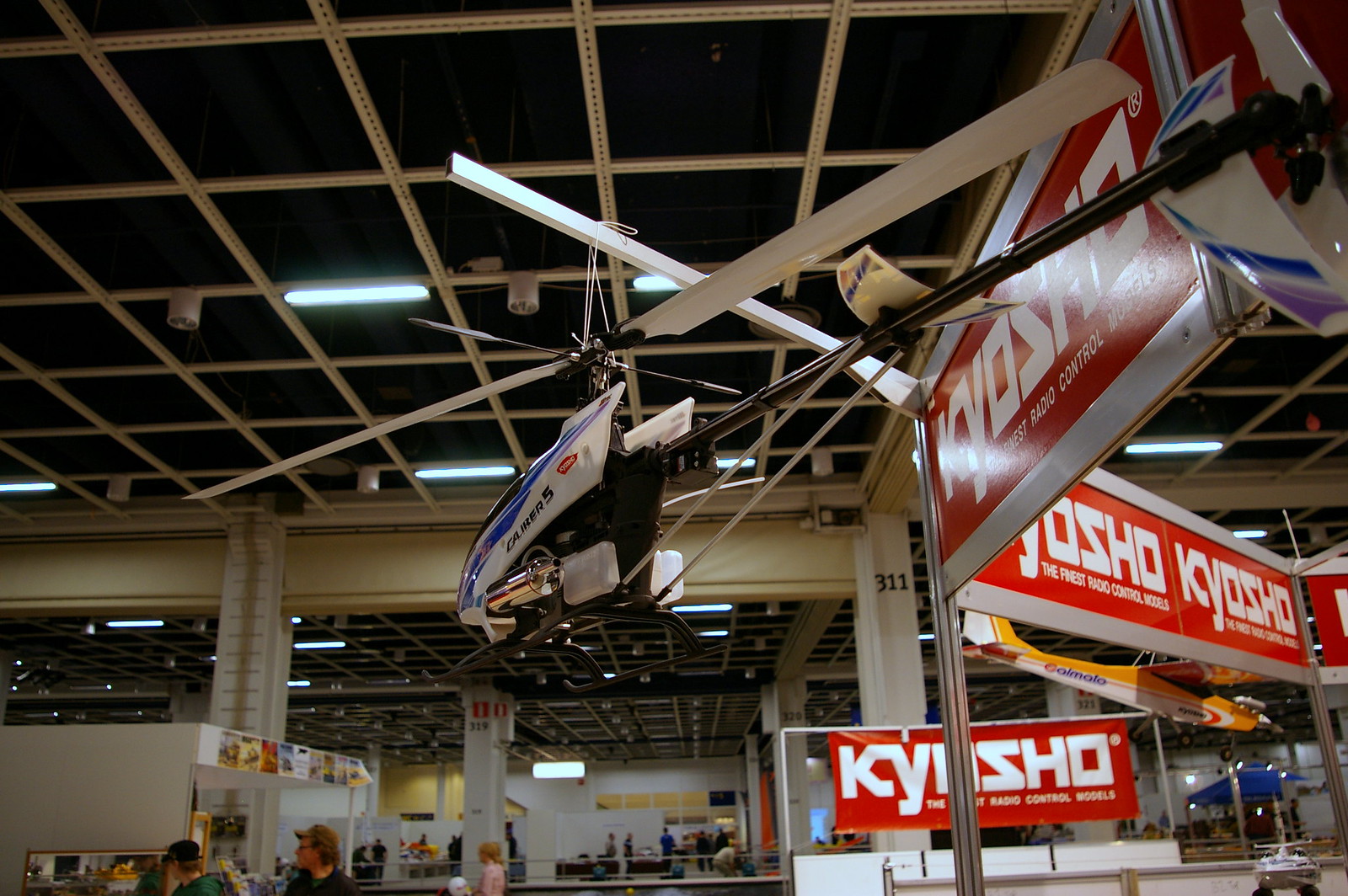In a large, warehouse-like store or convention center, a detailed display of a blue and white remote control helicopter is showcased prominently from the ceiling. The camera angle looks up, capturing the vast, dark-colored roof with a beige crisscross pattern. The helicopter, which features delicate, thin propeller blades and a seemingly flimsy build, hangs from a white or steel-colored rod. Nearby, three distinct red banners with "Kyosho" written in white letters add a splash of color to the scene. In the background, partially concealed, another model, possibly an airplane, is visible. The lower part of the image includes glimpses of people's heads, white columns, and various numbers, suggesting a busy and structured environment.